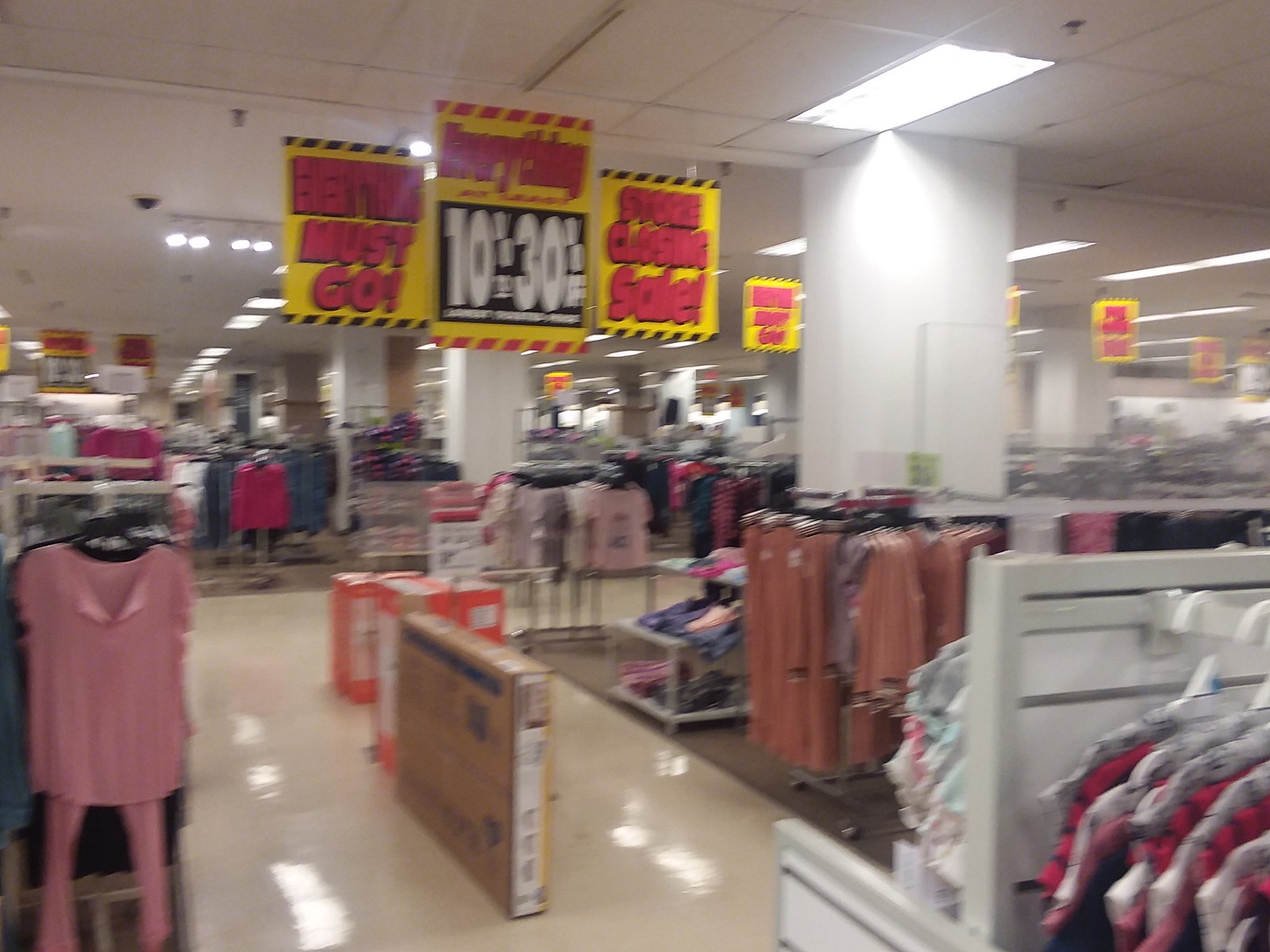In this image from a department store, a series of vibrant paperboard signs hang prominently from the ceiling, capturing immediate attention. The signs are designed in striking yellow, red, and black colors. The first sign, featuring bold red bubble letters, declares "Everything Must Go." Adjacent to it, another sign announces enticing discounts of "10% to 30% Off." Adding to the sense of urgency, a third sign proclaims "Store Closing Now."

On the store floor below, various clothing racks display a wide assortment of garments. Centrally located, a large square cardboard box stands out, containing a pinkish outfit which includes a short-sleeved top and long pants. Strewn around are additional items of clothing, contributing to the bustling and slightly disorganized atmosphere typical of a store in its final days.